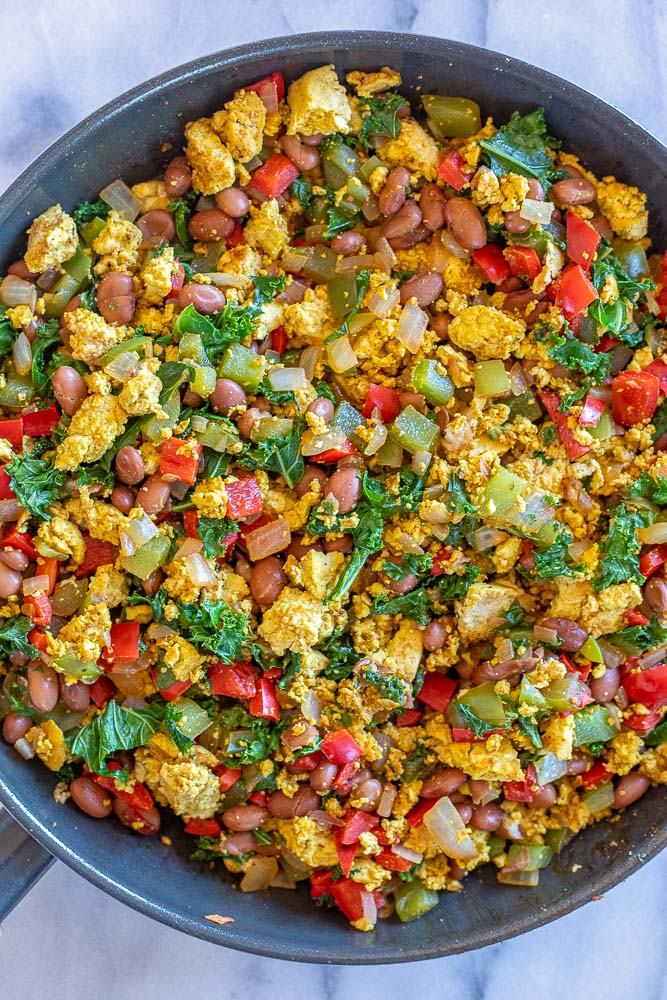A close-up image showcases a vibrant bean salad in a blue pot. The pot, partially cut off at the left and right, rests on a white and blue marbled countertop. The salad features an assortment of ingredients, including brown beans, chopped red tomatoes, green leafy vegetables, possibly kale or basil, and small translucent pieces resembling onion or cucumber. Yellow chunks, which might be scrambled egg, tofu, or a yellowish vegetable, add a pop of color. Light green celery bits and what appears to be white cheese, possibly parmesan, are also sprinkled throughout the dish. The backdrop of the scene includes a sky filled with clouds, with small patches of blue visible.